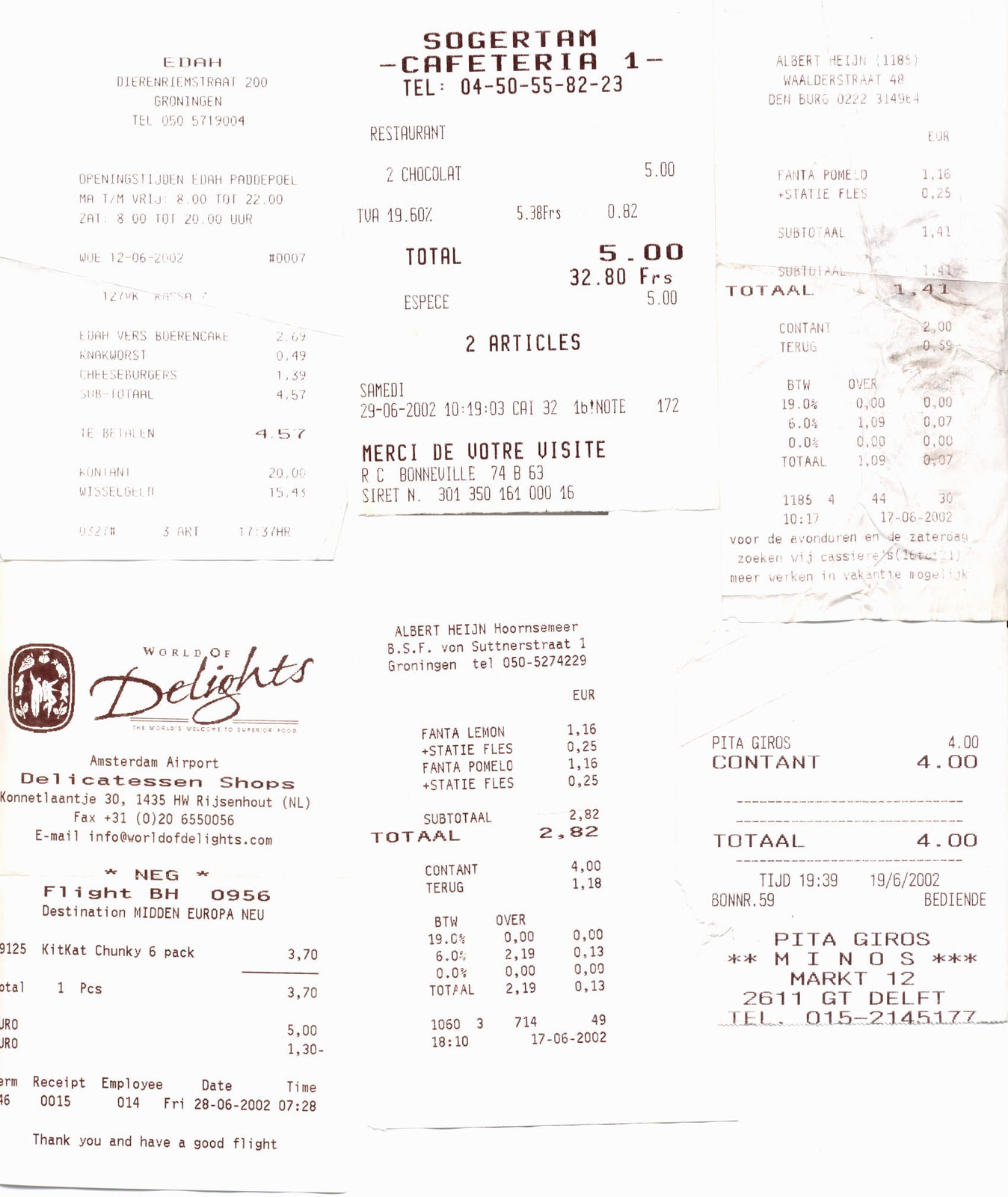The image displays six receipts, seemingly photocopied onto a single page and aligned next to each other. The receipts are in a foreign language and appear to be in black and white. The top left receipt is from a place called EDAH, although it's difficult to decipher the text. Next to it, the top right receipt appears to total around $4.00, though the details are distorted and unreadable. Below, the middle receipt showcases the name "Sol Ritam Cafeteria," or possibly "Soguntum Cafeteria," and lists an item described as "restaurant to chocolates" priced at $5.00. A telephone number, 04-50-55-82-23, is also visible. The remaining middle receipts include one labeled Albert, though specific details and numbers are unclear, and another potentially titled "Albert Hygen Horn Smear," both of which are not in English. The bottom left receipt clearly reads "World of Delights" and is inferred to be from a delicatessen shop. Adjacent to it on the right, the bottom receipt states "Pitajaros," with a total of $4.00 or slightly more. The receipts might be in Euros or Francs, leading to a possible origin in a European region, potentially the Amsterdam area, as indicated by the mention of "Delight, Amsterdam Airport."